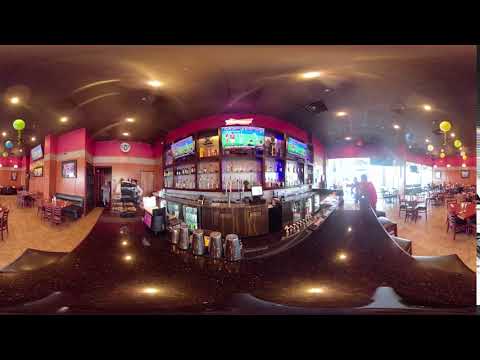The image captures the interior of a well-lit bar located inside a restaurant, taken from the viewpoint of someone seated at the bar counter. The expansive bar, which dominates the center of the image, showcases an impressive collection of assorted bottles arranged on shelves behind the counter. Several TV screens mounted on the wall above the bar display a sporting event, likely a soccer match. 

To the left and right of the bar, the space opens up into dining areas with numerous tables and chairs. The majority of these tables are empty, but in the distance, particularly on the right side of the bar, there are a few groups of people seated. The ceiling is adorned with both recessed lights and floating balloons in yellow, green, and blue, adding a festive touch to the ambiance. 

The décor features brown floors and a ceiling with a dark pink trim along the top of the walls, followed by lighter beige and orange hues. Condiments and napkins are piled on the tables, which are equipped with chairs and bar stools. A long window in the background allows bright light to filter into the room, further enhancing the vibrant atmosphere.